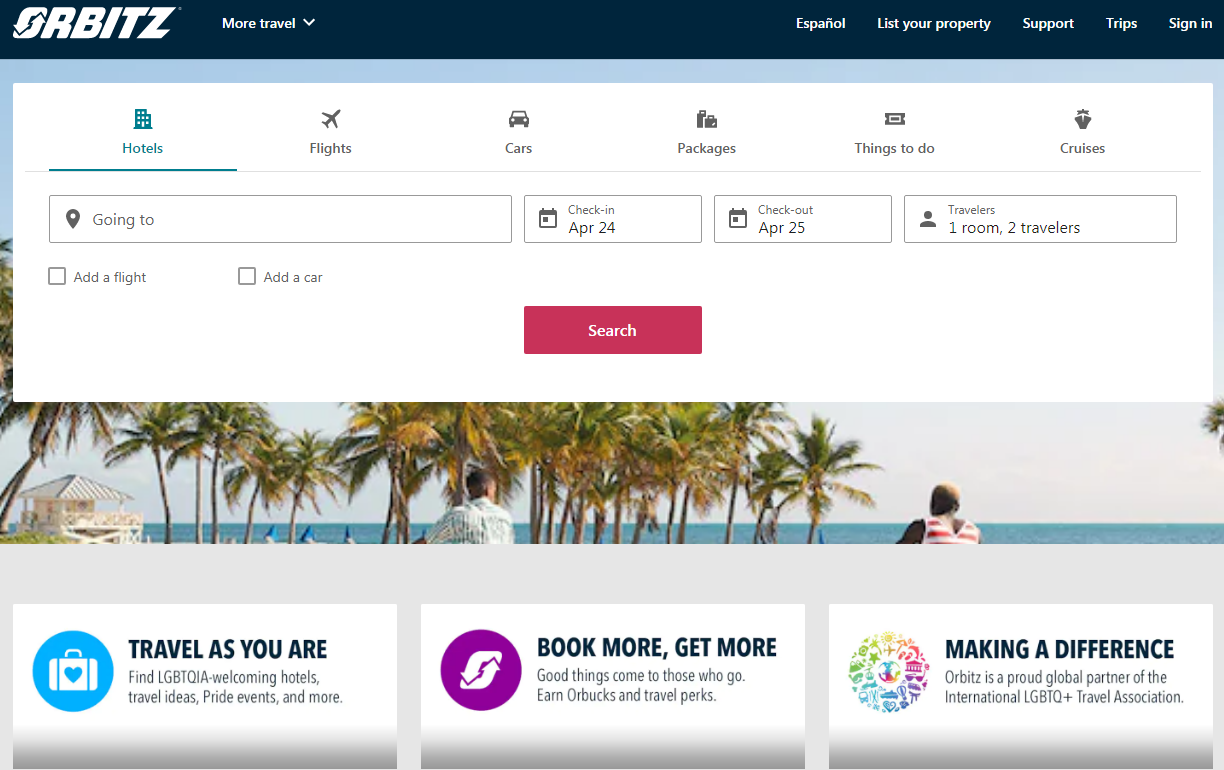The image is a screenshot of a travel website. At the top left, the website’s logo “Orbits” is prominently displayed. To the right of the logo, there is a section labeled "More Travel" with a down arrow indicating a drop-down menu. 

Adjacent to this are several navigation tabs listing various travel options: "Hotels," "Flights," "Cars," "Packages," "Things to Do," and "Cruises." On the left side of the page, there's a search bar labeled "Going to." 

To the right of this search bar, there are fields for "Check-in" (set to April 24th) and "Check-out" (set to April 25th), along with a dropdown for specifying the number of travelers which currently reads "One Room, Two Travelers."

Directly below these fields, there are optional selections for adding flight and car bookings, indicated by checkboxes labeled "Add a Flight" and "Add a Car." 

Centrally located on the page is a conspicuous "Search" button in white text against a magenta background. Below this button is an inviting image of an ocean setting with palm trees, suggesting a tropical destination.